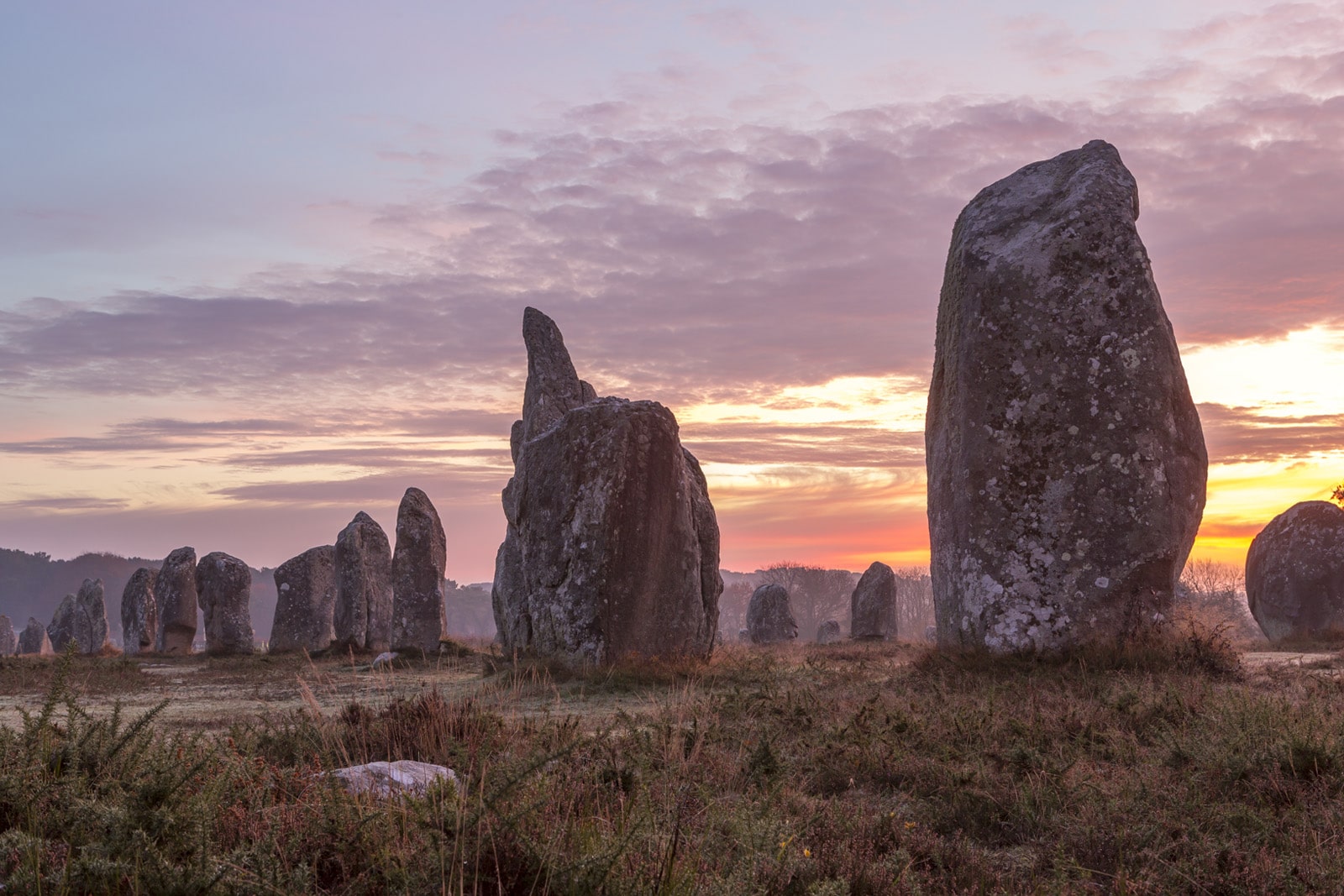The image captures the ethereal beauty of an ancient site, evocative of Stonehenge, set against a stunning early morning or sunset sky. The scene is dominated by strategically placed, towering rock formations that form two rows of jagged pillars stretching from the mid-left to the mid-right of the frame. These intentional structures stand majestically on a barren, desert-like plain punctuated by sparse, dried-up grasses and desert vegetation. The sky, transitioning from warm gold and pink near the horizon to streaks of purplish-gray clouds and blue, enhances the mystical ambiance of the landscape. Off to the right, the sun hovers low on the horizon, casting soft, warm hues that bathe the rocks in a golden glow. In the very faint background, a hint of woods with the outline of trees suggests a transition from the arid terrain. The scene is serene and devoid of people or animals, allowing the ancient and monumental nature of the boulders to take center stage in this captivating, solitary vista.